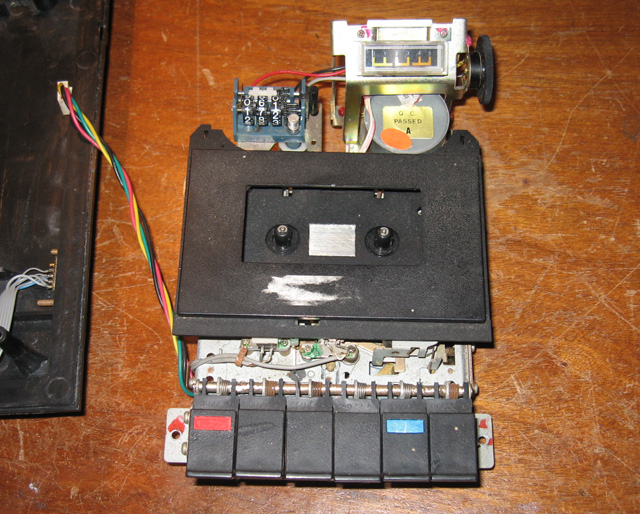The image shows a detailed photograph of a deconstructed tape recorder laid out on a scratched, medium brown wooden table. At the center of the image is the exposed slot for an audio cassette tape, flanked by two circular spools designed to rotate the tape inside its plastic casing. Above this, a mechanical counter with three spinning number wheels is visible, connected to other components by colorful wires.

Below the cassette slot lies the circuit board, coupled with a set of vertical black buttons—six in total. The leftmost button features a small red tab, while the second-to-last one has a blue tab. To the right side of the image, a metallic disc with a "QC Passed" gold sticker stands out, hinting at quality control testing. Surrounding these elements are various wires and mechanical parts, suggesting thorough disassembly.

The table beneath the tape recorder parts is a marked, weathered surface, adding a rustic backdrop to the scene. On the left side of the image, a dark brown rectangular object, possibly part of the device's electronic framework, completes the composition of this vintage audio equipment dissection.